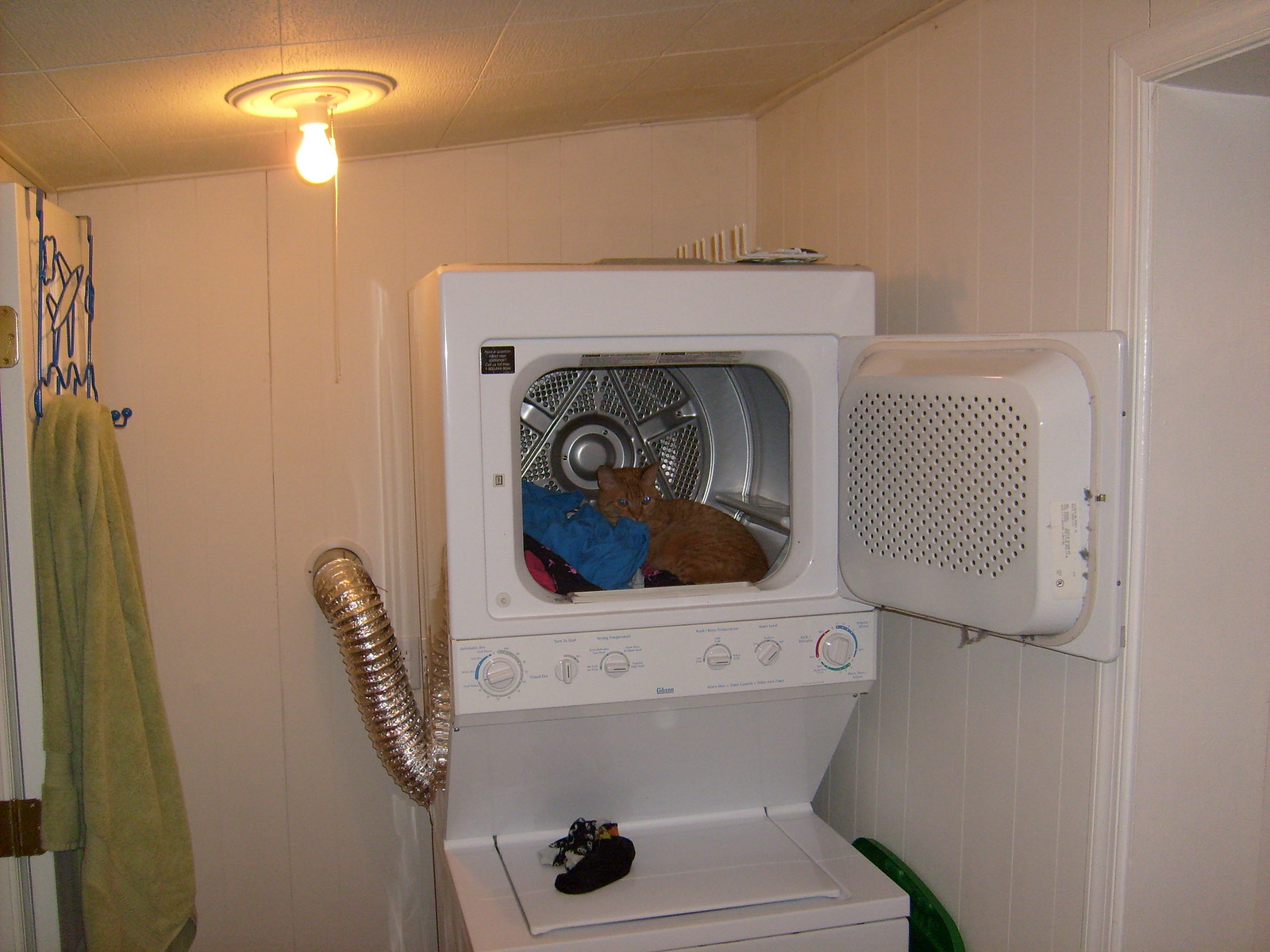This vividly detailed color photograph captures an interior view of a laundry room in a landscape orientation. The main focus is a stackable washer-dryer unit positioned directly in front of the viewer. The white dryer, perched above the washer, has its door open to the right, revealing a stainless steel drum partially filled with clothes and an orange tabby cat resting comfortably inside. The cat, with its eyes open and gazing into the distance, appears to have jumped in after the laundry was done, enjoying the lingering warmth. Below the dryer, the closed lid of the white washing machine is visible, with a few objects placed on top of it. Behind these machines, a hose and a steel duct connect to the back wall, supplying water and venting the dryer. The room is illuminated by a single, exposed light bulb hanging from the ceiling, casting a stark light that emphasizes the realism of the scene. Additionally, a green towel hangs on a metal hook affixed to the left wall, adding a touch of color and texture to the utilitarian space.